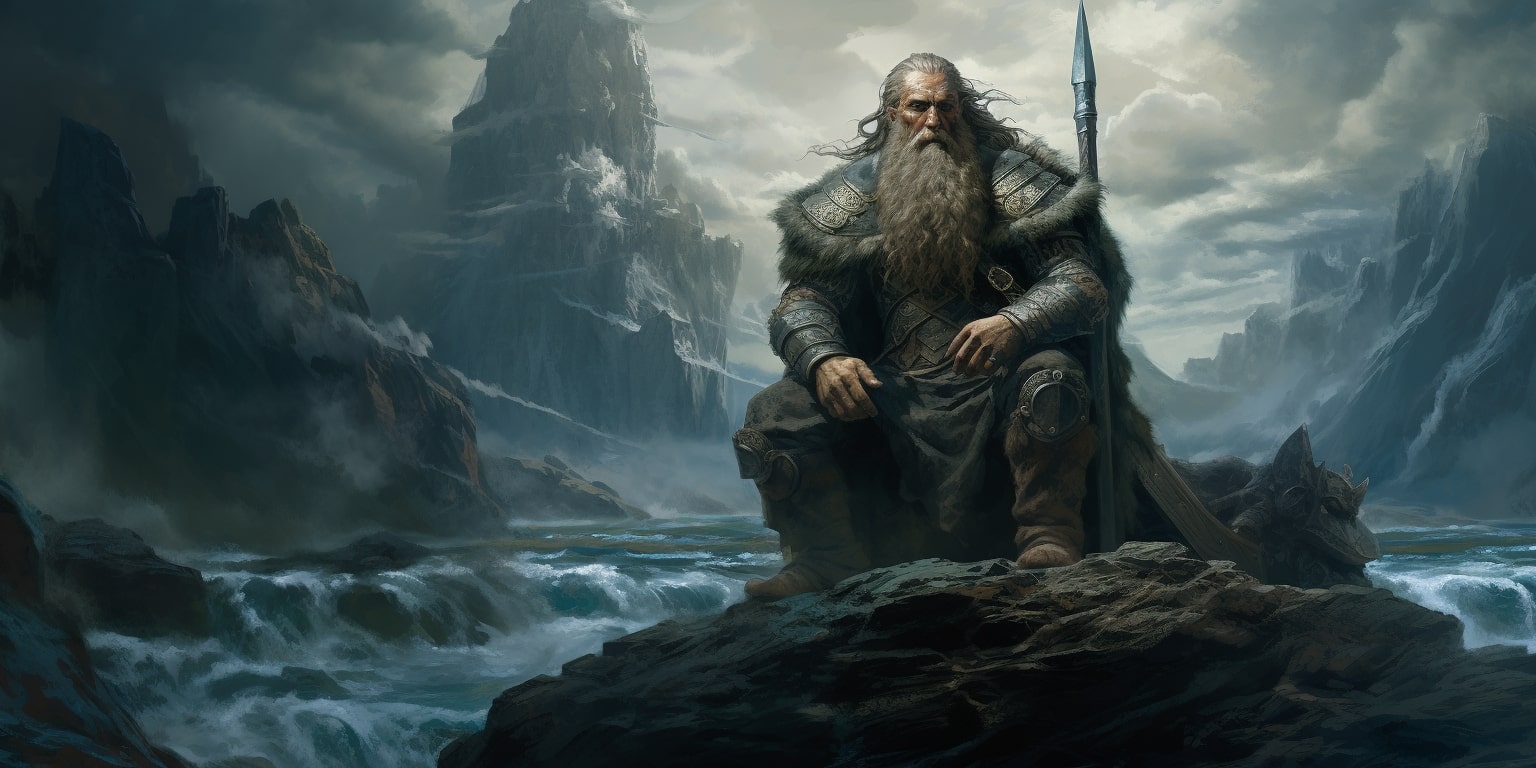The image depicts a powerful, wizard-like man with a long white beard and flowing hair, kneeling on a jagged rock amidst turbulent waters. Enveloped by stormy, darkened skies, the scene feels like a frame from an epic fantasy saga. The man is garbed in a leather cloak adorned with metal shoulder pads that are bordered with fur, and he wears metal gauntlets and boots, exuding an aura of medieval strength. His arms rest on his knees, hands closed in fists, and beside him stands a tall, sharp spear. Behind him, the rough waters churn vigorously, illuminated faintly by a break in the clouds. In the distance, a towering, castle-like structure looms, enhancing the mystical, foreboding atmosphere. The overall composition, with its grayish color palette and rugged backdrop of mountains and rocks, evokes a sense of ancient, fantastical landscapes often seen in works akin to "Game of Thrones."